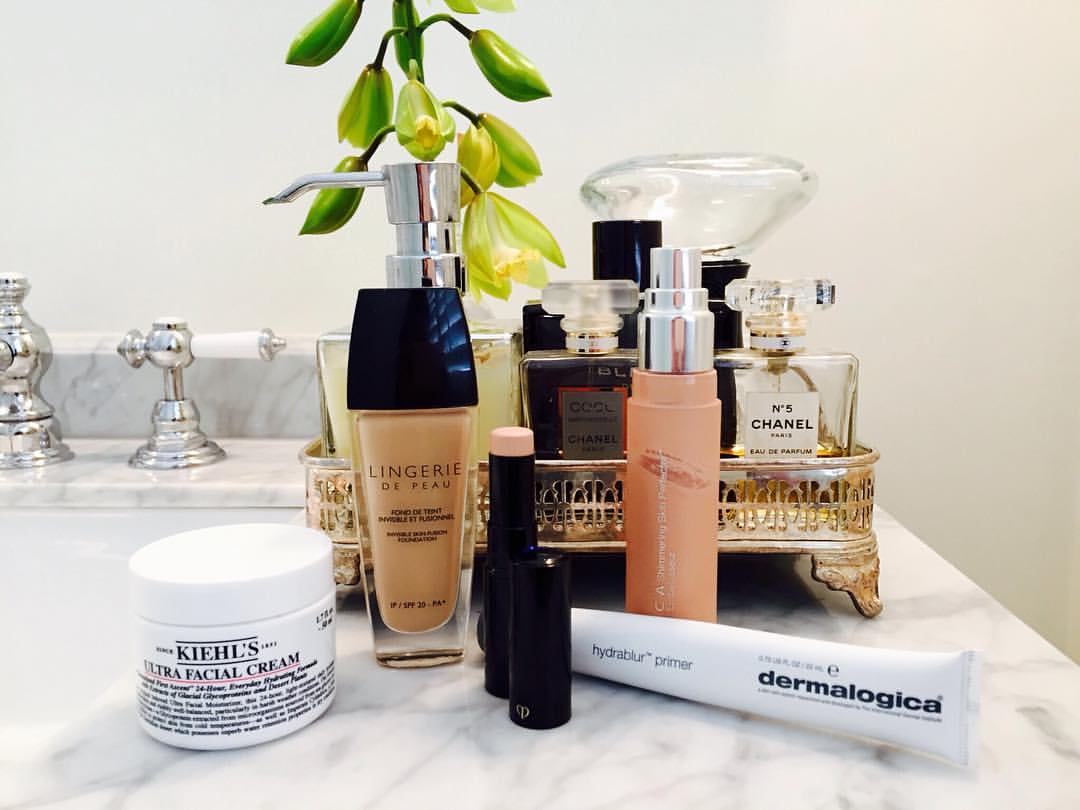A luxurious bathroom countertop is adorned with a curated selection of high-end beauty and skincare products. The marble surface glistens under the soft lighting, reflecting the opulence of the items displayed. Prominently placed is a white tub of Kiehl's Ultra Facial Cream, a coveted staple for radiant skin. Next to it, a sleek glass bottle filled with a rich brown liquid labeled "Lingerie de Peau" adds an air of sophistication. Lying nearby, a long white tube of Dermalogica promises professional-grade skincare. Behind these treasures sits an elegant golden tray, neatly organized with a range of luxurious perfumes, including the iconic No. 5 by Chanel and Kuhl by Chanel. To the back left, the chrome handles of the sink peek into view, complemented by a large chrome pump on another exquisite beauty product, tying together this lavish tableau of luxury and sophistication.